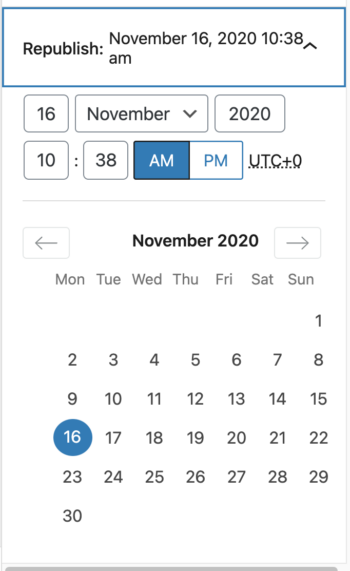This is an image of a mobile phone screenshot displaying a calendar entry interface. At the top, a white rectangle outlined in blue features the text "Republish" followed by the date "November 16th, 2020," and the time "10:38 AM." Below this, various input fields and controls are presented. The first row includes "16," "November" next to a downward arrow indicating a dropdown for month selection, and "2020." Directly beneath "16," the time is broken into "10" and "38" in two separate rectangles. The "AM" option is highlighted with white text on a blue background, while the adjacent "PM" shows blue text on a white background outlined in blue. To the right, "UTC +0" is underlined with a dotted line.

Beneath these details, the monthly calendar is displayed with arrows for navigating to the previous month (October) and the next month (December). The heading "November 2020" is followed by a week layout marked with the days "Monday, Tuesday, Wednesday, Thursday, Friday, Saturday, Sunday." The date "16" is circled in blue, indicating the selected day.